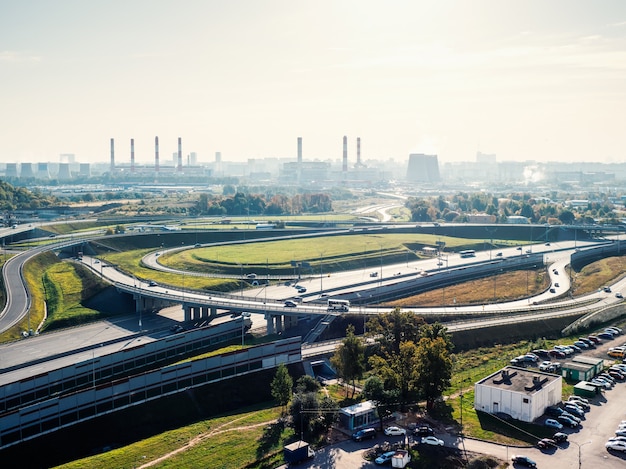This aerial photograph reveals a sprawling cityscape dominated by a complex highway system with multiple on and off ramps, some forming intricate, snake-like patterns. In the foreground, a parking lot full of cars and small white structures is nestled in an industrial area. Beneath an overpass, train tracks weave through the scene, with a train visible on the tracks. Mid-shot, various highways intersect with a modest amount of vehicular traffic, including some buses. The background stretches into a hazy horizon where a large power plant with tall smokestacks and large exhaust flumes stands prominently. The sky, potentially laden with pollution or just dense clouds, casts a bloomy light over the entire scene. Scattered trees and patches of green grass add a touch of nature amidst the urban and industrial sprawl.